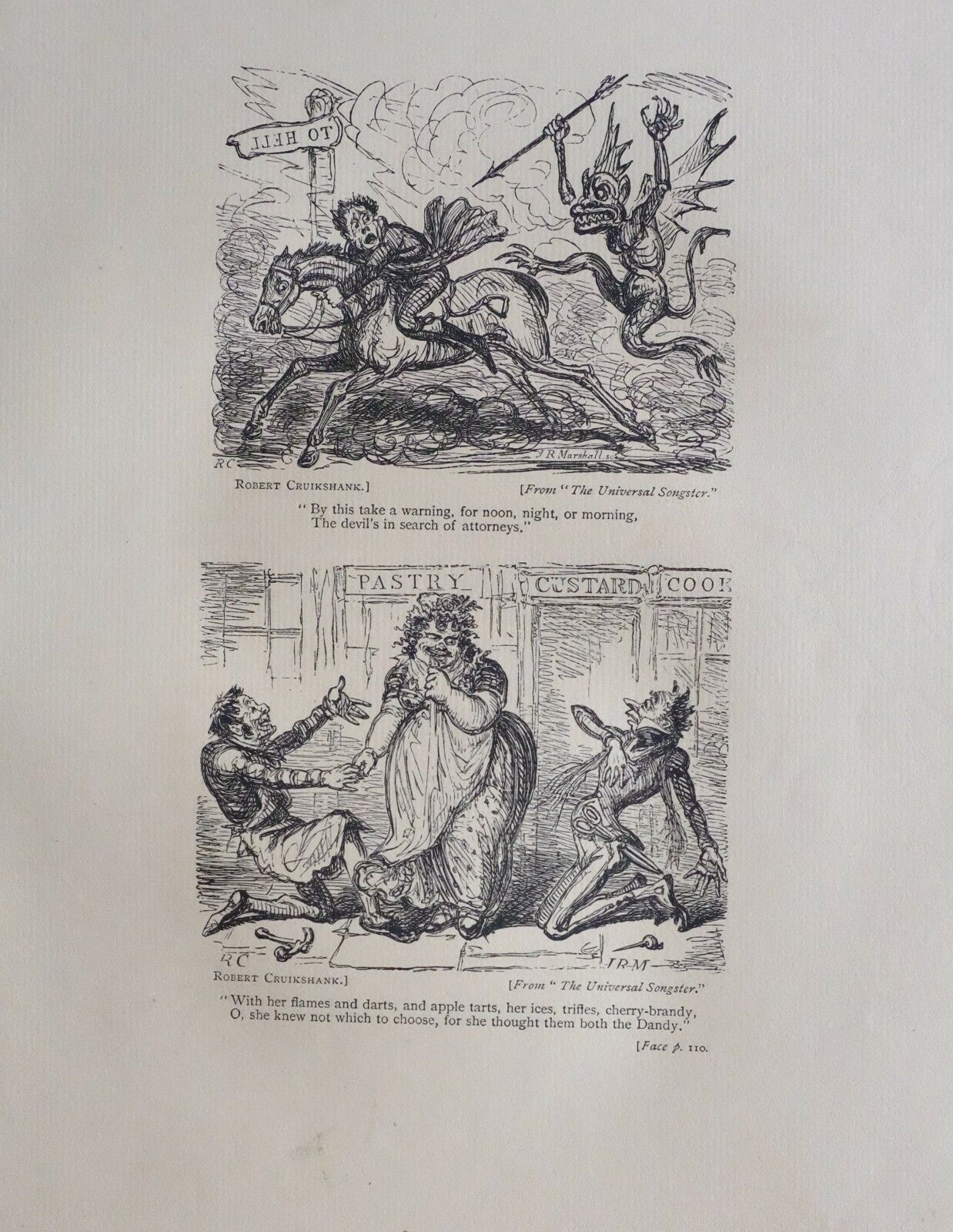The image is comprised of two black-and-white comic drawings, likely from a children's storybook or a satirical collection, set against a gray background.

The top drawing features a dramatic scene with a man riding a horse, looking very scared. The horse is positioned on the left, while a menacing dragon with sharp, spiky features, large wings, and prominent teeth is on the right, appearing to kick the horse with its legs flopped forward. The dragon holds an arrow and seems to have a signboard, clouds, and a forested backdrop behind it. The caption below reads: "By this, take a warning for noon, night, or morning. The devil is in search of attorneys," indicating a warning about lawyers, with the credited artist being Robert Cruikshank.

The lower drawing depicts a large, imposing woman standing in the middle, with two men on either side of her, both on their knees. One man is lying on the ground, holding her hand, while the other is also on the ground, staring up at her with a scared expression. In the background, there appears to be a shop sign advertising pastries, custards, and cookies. Scattered on the floor are a hammer and nail. The caption below this drawing is whimsical: "With her flames and darts and apple tarts, her eyes are trebles and cherry hand brandy. Oh, she knew not which to choose, for she fought them both to dandy." This, too, is credited to Robert Cruikshank.